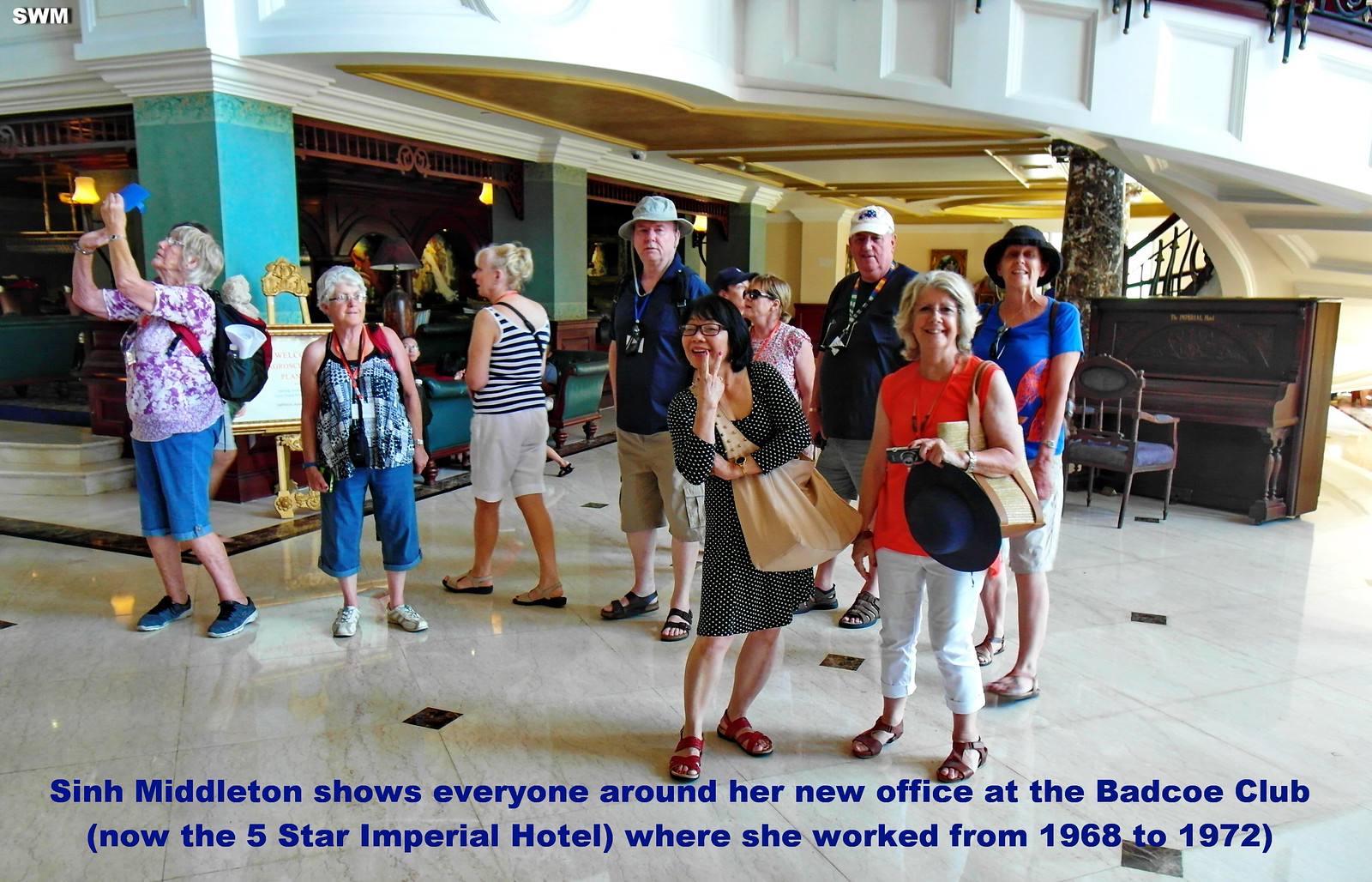In this detailed photograph, a group of approximately nine to ten elderly individuals is gathered, most likely in the lobby of a hotel. They appear to be on a guided tour with Sin Middleton, who is showing them around what is now the five-star Imperial Hotel, formerly known as the Badco Club, where she worked between 1968 and 1972. The lobby setting is elegantly designed, featuring tile floors, turquoise pillars, a grand piano in the background, and a spiral staircase. The group, comprised of both men and women, with the men donning baseball and regular hats and the women in summery attire, seems to be a mix of individuals both posing for the photograph and casually exploring their surroundings. The caption below the image, written in blue text, reads: "Sin Middleton shows everyone around her new office at the Beto Club, now the five-star Imperial Hotel where she worked from 1968 to 1972."